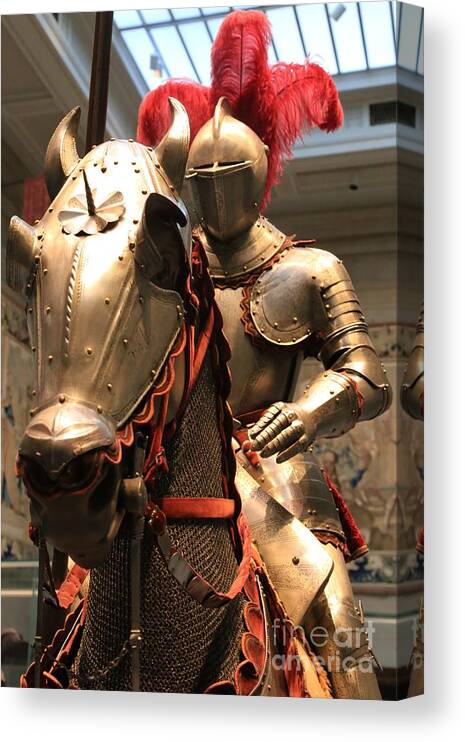This detailed canvas print features an intricate photograph of a knight in ornate armor, astride a realistically rendered mannequin horse, both situated in what appears to be a museum setting. The knight's armor shines in a metallic silver color with slightly reflective surfaces. The pauldrons curve near the top right of the frame, transitioning into segmented arm pieces ending in angular gauntlets that flare out at the rear. The helmet, predominantly smooth with a single flange on top, has a shallowly pointed front with two menacing black eye slits. Emerging from the helmet are three large red plumes - one vertical and two drooping to either side. 

The horse mannequin is equally armored, featuring a similar metallic material. Its headpiece sports a floral pattern between the eyes, accented with a central sharp point and two lateral horns, each accompanied by flares above the eyes. Beneath the head, the tall neck is draped with chainmail, bordered by red leather flanges around the neck base and the horse's helmet bottom. Additional red leather straps and harnesses zigzag across the armor, adding visual depth. 

In the backdrop, an ornate beige wall adorned with blue and white paintings is blurred, giving a sense of depth. From the ceiling, a window lets in a soft whitish-blue light, enhancing the ambiance. The bottom right corner of the canvas carries a faint white watermark reading "Fine Art America." The image itself is printed on a canvas giving it a 3D appearance, with slight leftward tilt revealing the right edge of the print continuing over the sides, offering a striking, immersive perspective.